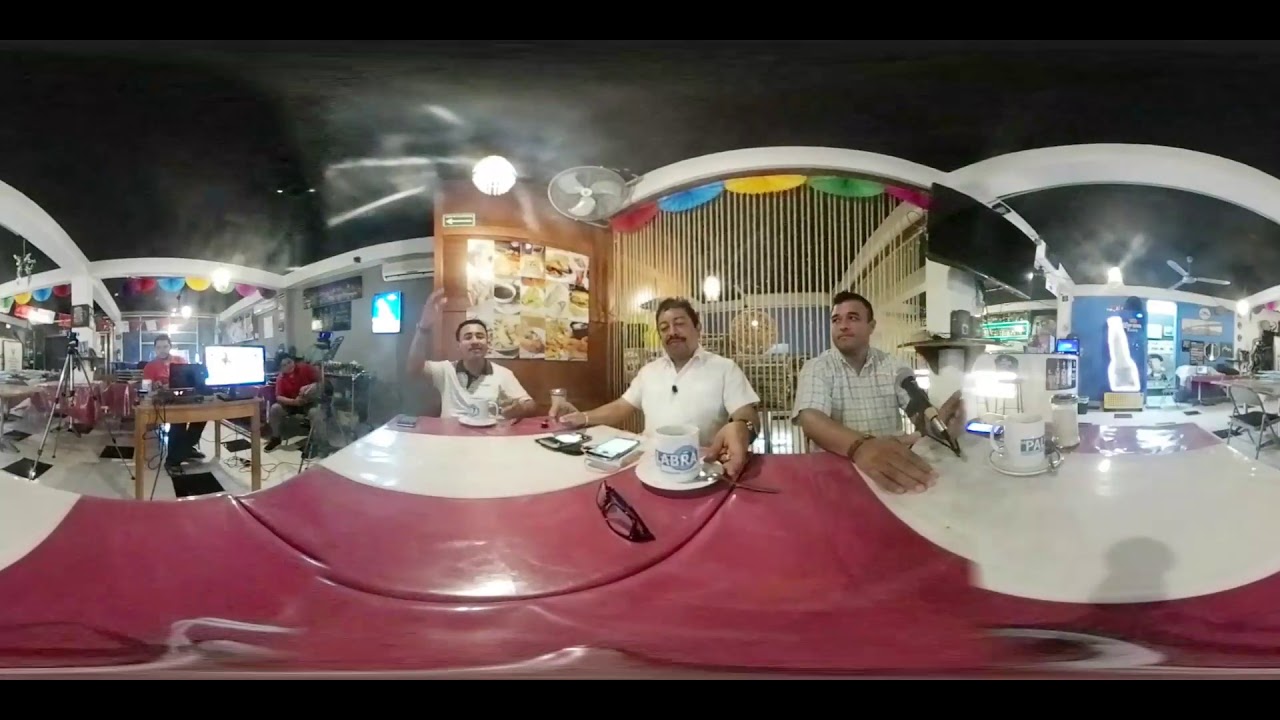In this bustling, multi-faceted scene, three Hispanic men are seated at a prominently red and white table, possibly made of plastic or marble, at an event or public space that resembles a mall. Each man is dressed in short-sleeved shirts and is holding white coffee mugs; notably, the mug held by the man in the center bears the inscription "Labra." The man on the left has his right arm raised, while the man on the right speaks into a microphone, adding a dynamic aspect to their interactions. On the table in front of the central figure, there's a tablet, perhaps an iPad mini, along with folded glasses. The background reveals a busy environment with a slatted room divider, colorful semicircle valances, and several shopfronts. One shop has a menu with pictures of food, another appears to be closed with a gate down, and a third is adorned with blue elements featuring a large bottle image. Additionally, there's a fan positioned between two shops on the upper left, and a neon figure behind a table and chair on the right. Despite the chaotic and overlapping circular frame of the image, suggesting a scalloped or binocular-like view, the scene is saturated with vibrant colors and lively ambiance.